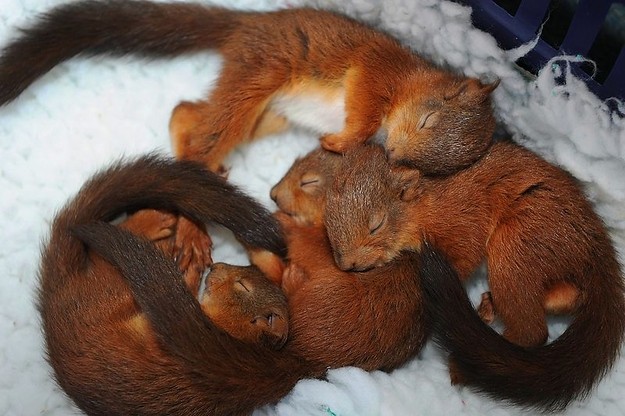In the image, we see four young red squirrels nestled closely together as they sleep on a white, fluffy textile. The squirrels have reddish-brown fur, with darker brown tails resembling that of a fox, and they all share white bellies tinged with a slight yellowish hue. Their small ears and closed eyes add to their peaceful appearance. They are arranged in the center of the image, with part of the top right corner showing a dark bluish crib that seems to hold this cozy scene.

The squirrel positioned at the top of the image sleeps with its body facing downward and its head resting on the body of the squirrel at the bottom right. The middle squirrel, partly covered by its siblings, curls up tightly in a ball with its eyes closed, creating a sense of closeness and warmth. To the left of this central squirrel, another one nestles with its head resting on the middle sibling’s back. Lastly, the bottom left squirrel curls up in a partial fetal position, adding to the overall affectionate tableau. The white textile beneath them appears soft and matted, providing a snug bed for the adorable quartet.